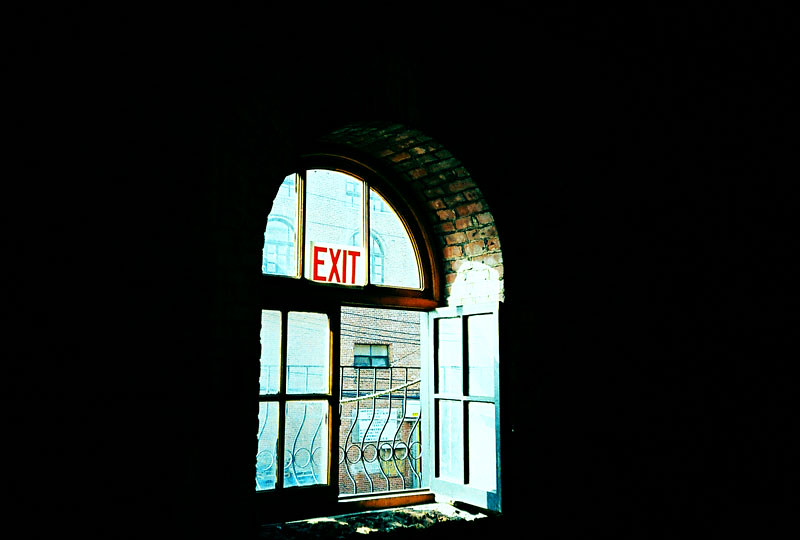In the dimly lit interior of a dark room, the focal point of the scene is a curved, column-like exit leading to a windowed door bathed in daylight. The door, which swings inward, features four glass panes, though it's partially obscured and could possibly be double doors. A prominent, large red exit sign dominates the lower half of the middle window. An older rug lies in the doorway, leading to an ornate black railing just outside. This railing serves as a protective barrier. The view through the bright windows reveals the exterior of a nearby brick building with black windows, indicating the observer is not at ground level. The room's darkness contrasts sharply with the daylight streaming in, emphasizing the exit as the main source of light.